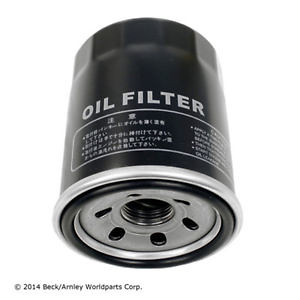This image captures a close-up, top view of a black cylindrical oil filter. The filter features light gray capitalized text on its smooth surface, clearly stating "OIL FILTER." Below this text, there is a rectangular label with rounded edges, containing a mix of Asian characters and English text, primarily in white, denoting specifications likely in Japanese or Chinese. The bottom of the filter is silver, outlined by a black ring. There are six holes symmetrically placed around a central, screw-threaded hole on the bottom surface. The background is white, contrasting with the dark filter. Additionally, at the very bottom of the image, the copyright "©2014 Beck/Arnley World Parts Corp." is printed, indicating the year and ownership of the image.